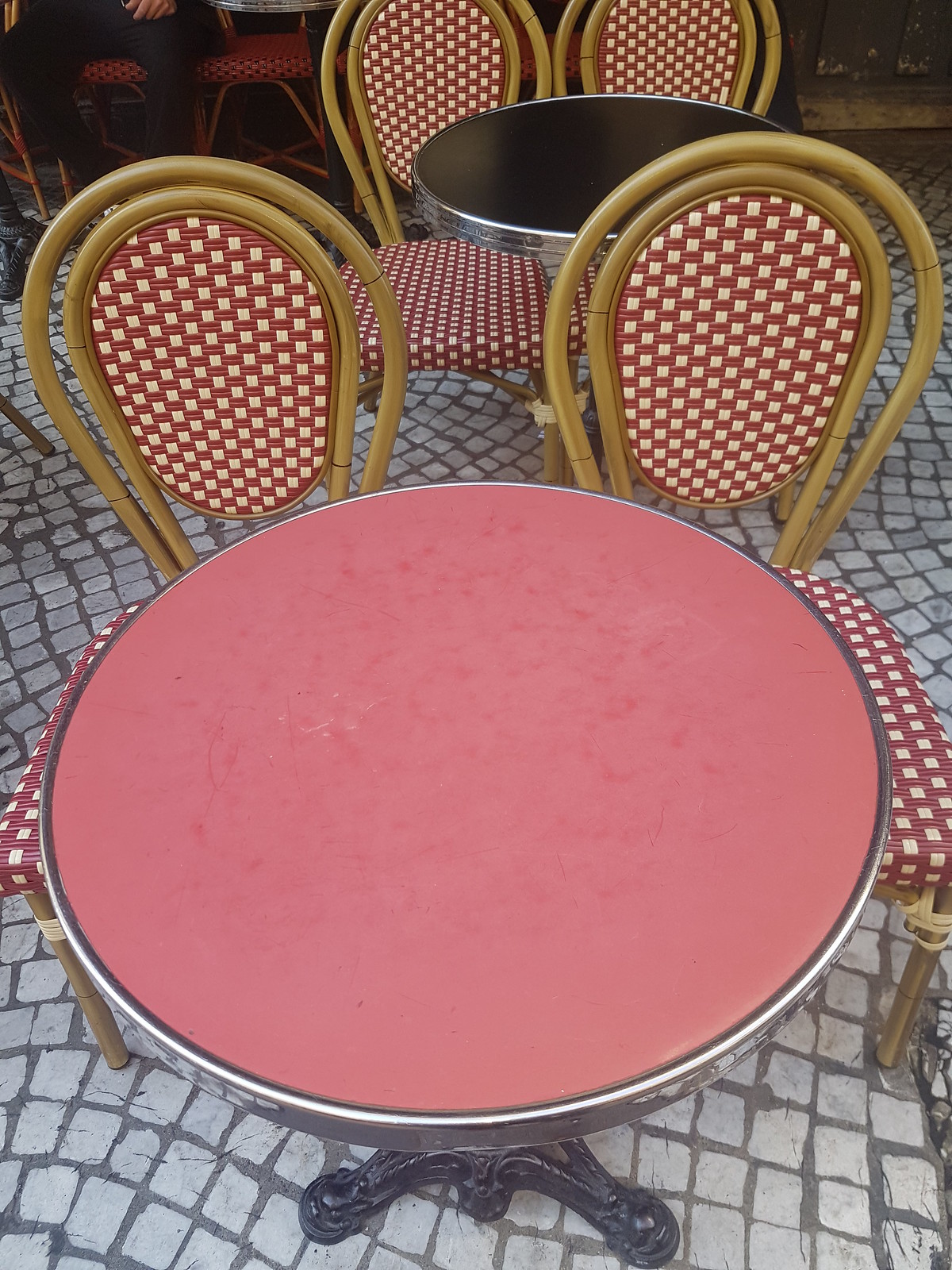This image features a pair of tables situated on a floor of small gray bricks, viewed from above. The central and most prominent table has a peach-colored top with a silver metal edge and a black metal base, complete with visible metal feet arranged in a stabilizing configuration, possibly with a third leg obscured from view. Two light brown wooden chairs with rounded backs are placed behind this table, each adorned with a red and white polka dot checkerboard patterned seat and backrest. Another table in the background has a similar design but distinguishes itself with a black top and the same silver metal rim. Accompanying this table are two identical chairs with the same red and white polka dot checkerboard pattern. In the far background, additional chairs of the same style can be seen, along with a partially visible person seated on one of them. The flooring, made of small gray stone tiles with gray cement in between, further enhances the detailed ambiance of the setting.